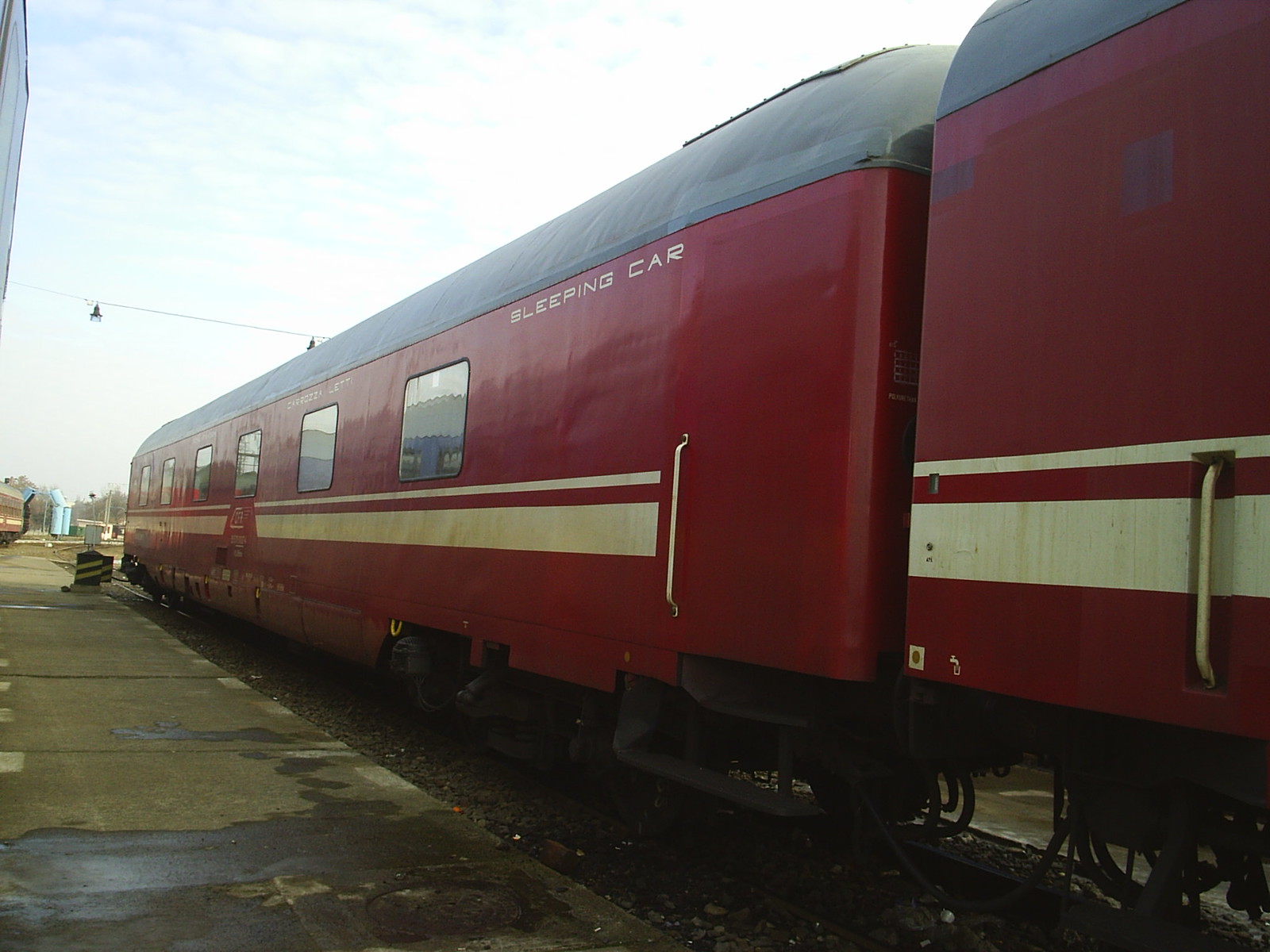This detailed color photograph captures an old red train on the tracks, prominently featuring a long, red sleeping car. The car has a grayish-black roof and a striking gold stripe that runs along its side, punctuated by six large windows. The text "sleeping car" is written in white near the top edge of this car. The train is angled diagonally from the right edge of the photo towards the left, and a second car, similarly colored with a gray roof and gold stripe, is partially visible attached behind the sleeping car. In the foreground, the train sits next to a brownish sidewalk, and a large wet spot is evident on the ground nearby. The background presents a mix of blue towers and trees in the distance under a sky filled with grayish-blue clouds, creating an overcast atmosphere with much white cloud coverage. The overall scene appears devoid of people, suggesting a tranquil yet historic moment captured with vivid detail.